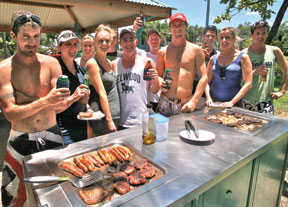The image captures a lively summertime barbeque with approximately 12 friends and family members, a mix of men and women enjoying the sunny day. Many are dressed in tank tops and short sleeves, with some men shirtless and wearing hats. The group, spread out from left to right, is positioned facing the camera and enjoying drinks in either cans or bottles. The barbeque station with its stainless steel top is active; hot dogs and hamburgers are being grilled, alongside other indiscernible items. Visible beside the grill, which also features a spatula, tongs, and a bottle of what seems to be olive oil, are empty Tupperware containers and cabinet doors beneath. A central table, covered by an umbrella, holds more meats. The setting includes palm trees, other greenery, and a covered pavilion in the background, enhancing the relaxed outdoor atmosphere. The vibrant colors within the photo include shades of brown, tan, red, black, green, blue, beige, and silver, portraying a vivid and inviting scene.